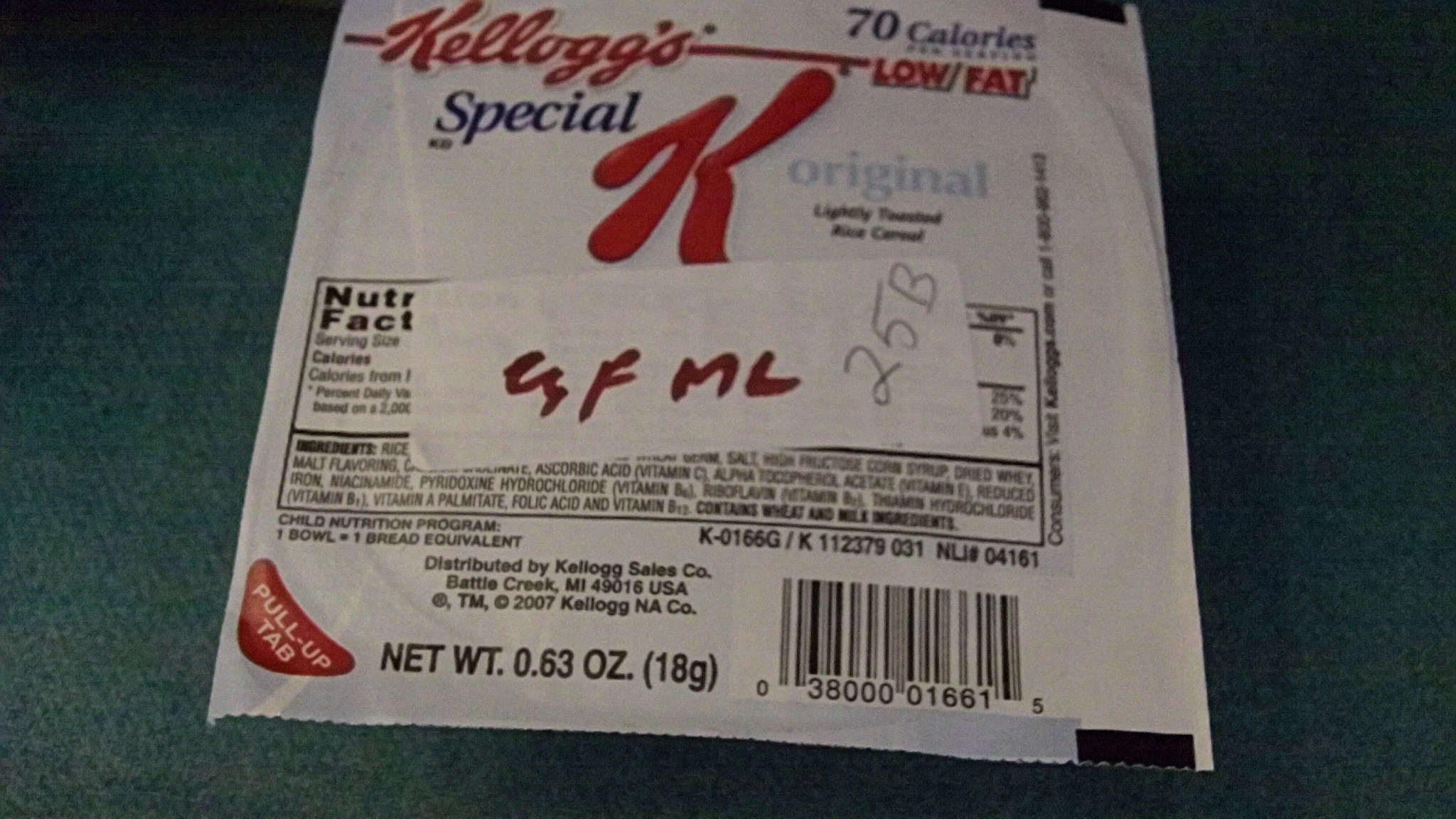This is a photograph of a plastic wrapper for Kellogg's Special K cereal. The predominantly white packaging features red lettering prominently displaying "Kellogg's Special K Original," along with a notation that each serving contains 70 calories and is low in fat. The wrapper includes standard nutritional facts, although they are partially obscured by a white sticker with red text that reads "FML 25B." The bottom of the wrapper has a pull tab for easy opening and indicates a net weight of 0.63 ounces (18 grams).